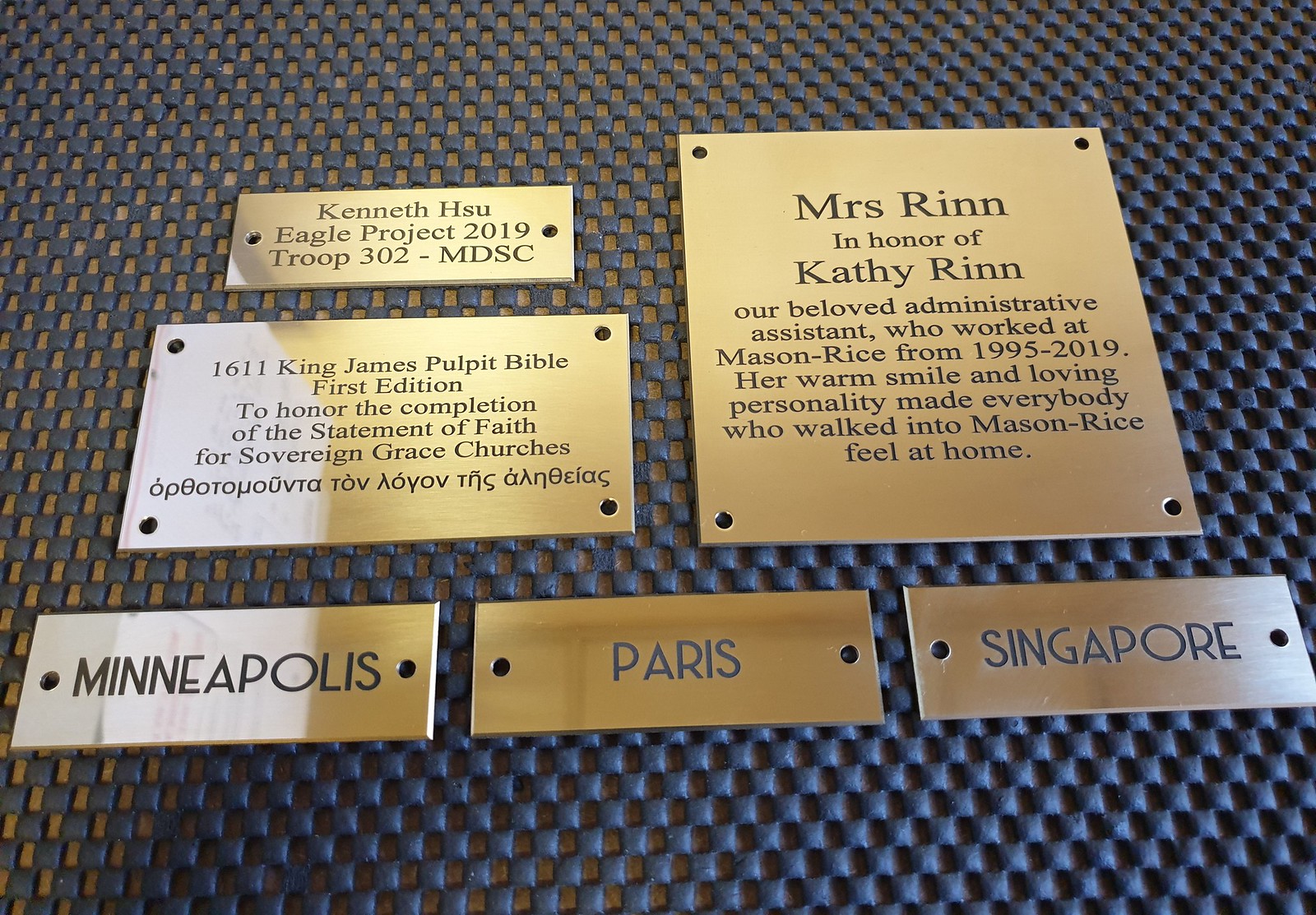The image displays a collection of engraved plaques, with a highly detailed and organized presentation set against a backdrop of alternating small blue-black and blue-cream squares, suggesting the blue squares are protruding elements while the cream squares form the base wall. In the foreground, several gold metallic plaques, arranged in a grid-like fashion, feature etched black inscriptions honoring various entities and people.

At the bottom of the arrangement, three rectangular plaques bear the names of cities: "Minneapolis," "Paris," and "Singapore." Each name stands out prominently in black on the brass-colored metal. 

To the left, two horizontally oriented plaques provide specific tributes. One mentions King James Public Bible First Edition, celebrating the completion of the Statement of Faith for Sovereign Grace Churches. The other smaller plaque reads: "Kenneth 2, Eagle Project 2019, Troop 302 MDSC."

On the right side, a vertically oriented plaque honors a notable individual: "Mrs. Wrynn," in recognition of Kathy Wrynn, a treasured administrative assistant at Mason Rice from 1995 to 2019. The text highlights her warm smile and loving personality, which made everyone feel at home.

The carefully arranged plaques, varying in size and message, collectively form an intricate display, likely intended to honor significant contributions and perhaps to showcase the craftsmanship of the engravers.